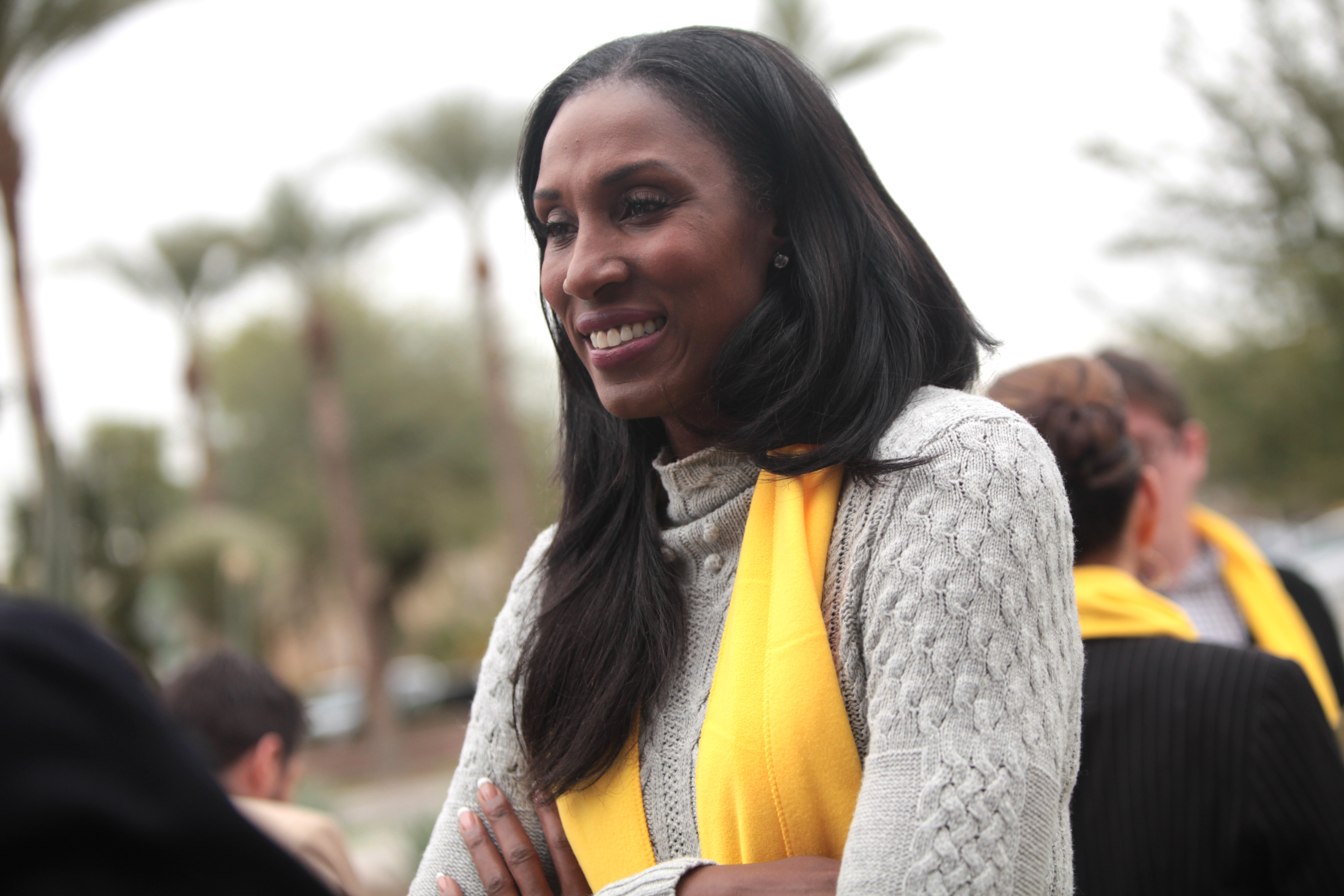The image features a smiling African-American sports journalist from ESPN, wearing a gray knitted sweater with a swirly braid pattern and a bright yellow scarf. She has long black hair worn down and sports an earring on her left ear, along with peach and white fingernails. Her arms are crossed in front of her. Behind her, the background is blurry but reveals several individuals—a woman in a black suit jacket with a yellow scarf similar to hers, a man in a black top also with a yellow scarf, and two other people, one with brown hair in a beige jacket. The scene is set amidst tall palm trees with a bright, mostly white sky, indicating it's daytime, likely overcast but pleasant enough for outdoor activities.